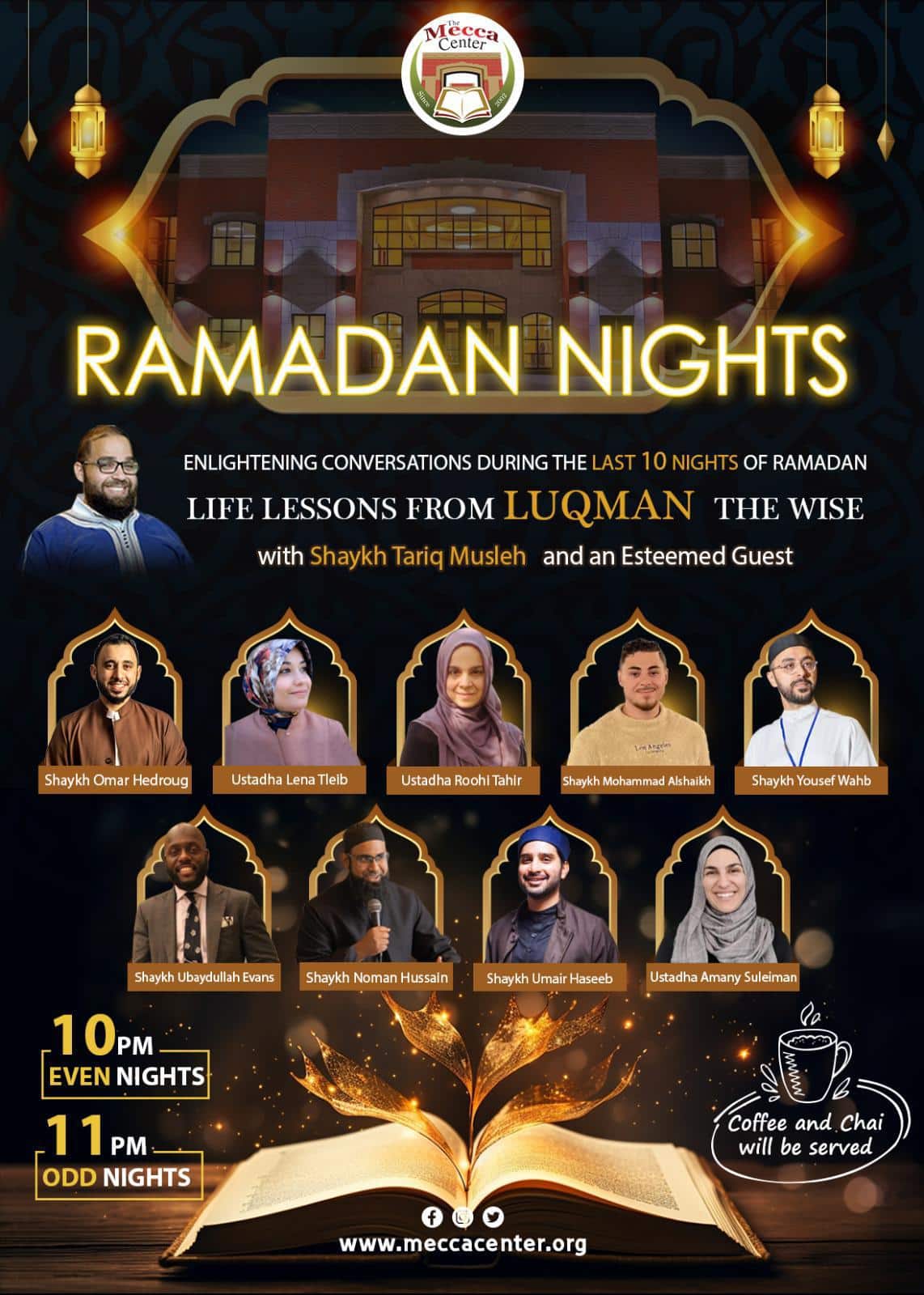The poster advertises an event titled "Ramadan Nights" in bright yellow neon letters, set against a black background adorned with decorative lights and diamond-shaped ornaments at the top left and right corners. Central to the image is a building and Mecca Center logo, both positioned in the top middle section. Below the title, the text reads, "Enlightening Conversations During the Last 10 Nights of Ramadan: Life Lessons from Luqman the Wise with Sheikh Tariq Musleh and an Esteemed Guest." Sheikh Tariq Musleh, depicted beside this text, sports a beard and glasses, dressed in a blue jacket with white or gray trim. 

Beneath this section are images of nine other guest speakers, arranged in two rows. The top row includes three males and two females, with Sheikh Omar Hadruk, Ustadh Lynn Taib, Ustadh Ruh Tahir, Sheikh Muhammad Al-Saud, and Sheikh Yusuf Wab among them. The bottom row features four individuals: three males and one female, all dressed in various shades of brown and purple, with the women wearing headdresses and the men either having dark brown hair or sporting black hats.

At the bottom of the poster, an open book with a golden leaf springing from it sits centrally, symbolizing the enlightening theme of the discussions. To the left, the poster details the event timings: "10 p.m. Even Nights" and "11 p.m. Odd Nights." The Mecca Center’s website, www.meccacenter.org, along with its Facebook, Instagram, and Twitter icons, appears slightly above this timing information. On the bottom right, an illustration of a steaming coffee cup accompanied by the text "Coffee and Chai will be Served" informs attendees of the available refreshments.